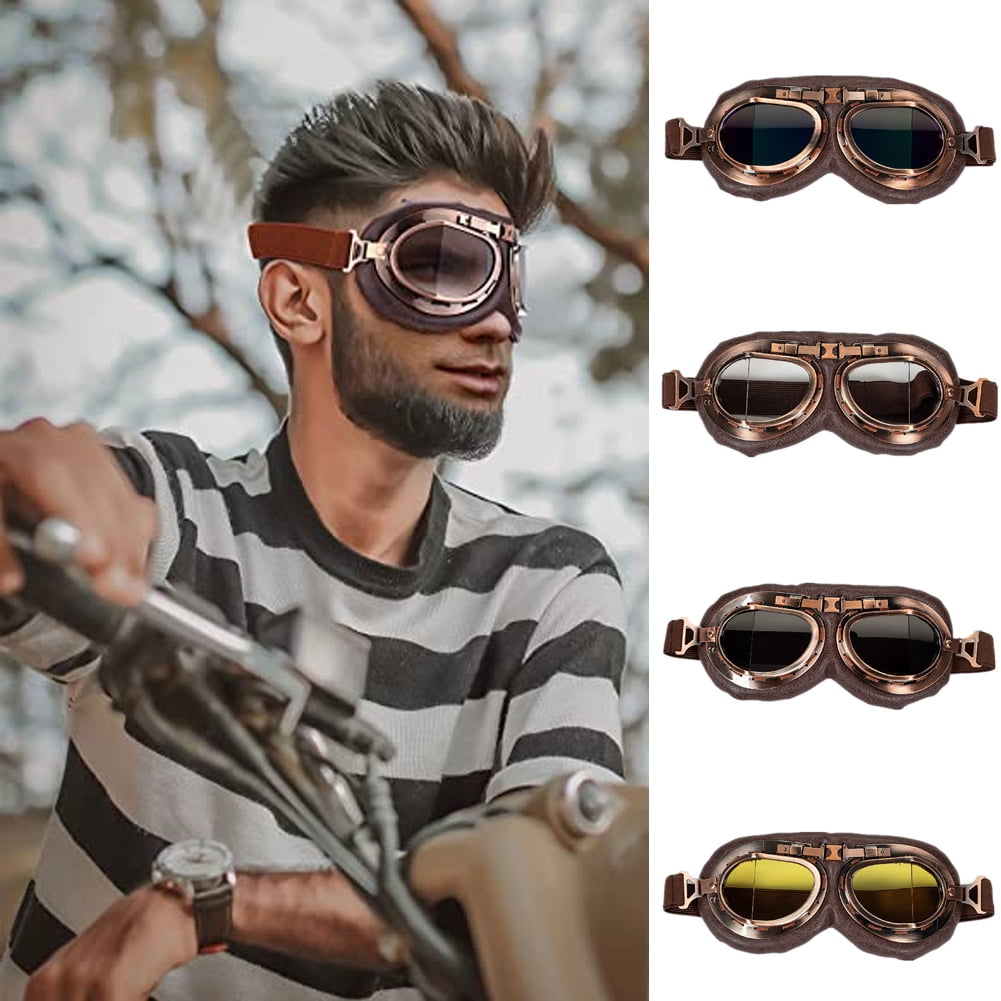In this dynamic product image, a bearded man with spiky brown hair is prominently featured against a blurred outdoor background of sky and trees. He exudes a confident aura, seated on a motorcycle and donning a white and gray striped t-shirt. His left hand grips the bike handle where the brake lever is typically situated, while his right arm rests casually on the bike's front fender, which is light brown in color. A large watch with a white face and what appears to be gold hands is visible on his wrist. On his face, he wears a pair of sleek, protective biking goggles.

To the right of this scene, four pairs of motorcycle goggles are displayed vertically against a white background, showcasing their various tints and finishes—from dark tinted lenses on the top three pairs to a yellowish tint on the bottom pair. These goggles, complete with straps for secure fitting, highlight the subtle variations in shading and style, emphasizing their functionality and stylish appeal for biking enthusiasts.